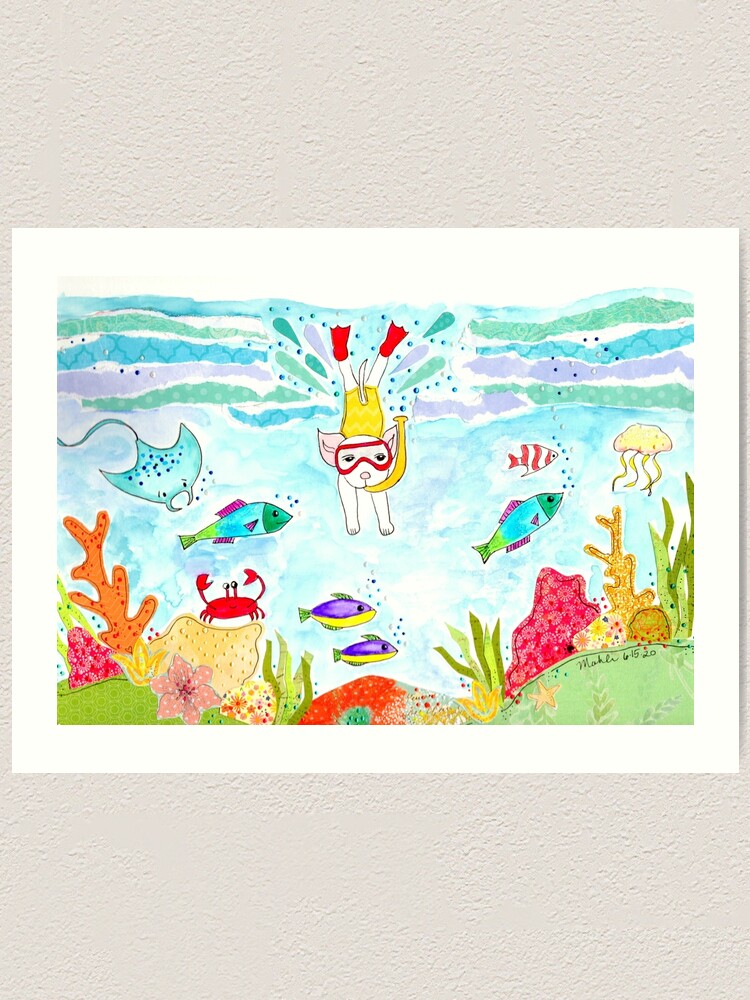The illustration, seemingly created with watercolor, depicts a charming underwater scene featuring a dog-like creature, which could also resemble a pig due to its pink ears and slightly ambiguous features. The creature, wearing yellow swimming trunks and red flippers on its back legs, is depicted diving beneath the water with a yellow snorkel in its mouth and red-rimmed goggles over its eyes. Its front paws are pointed downward while it faces the viewer, and its back legs splash above the water's surface, which is textured with greenish, bluish, and purple lines.

Surrounding the creature are various forms of marine life, including a stingray, a crab, and multiple fish. Notably, two fish below the creature are purple on top and yellow underneath. On the left side, there's a fish, a crab, and a stingray, while on the right, more fish and a jellyfish are visible at the far edge. The underwater environment is enriched with colorful plant life, featuring corals in shades of red, yellow, and green. The ocean's layers display a palette of light blue, green, turquoise, and purple hues, adding to the vibrant and whimsical atmosphere of the underwater adventure.